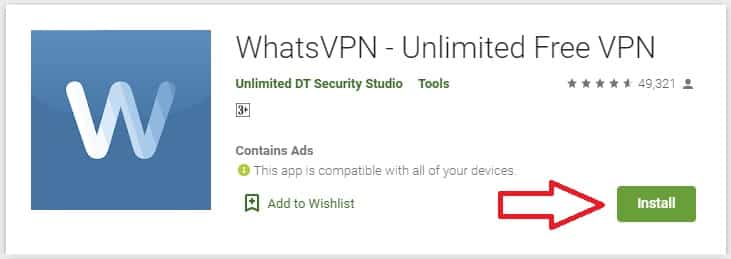The image is a promotional banner for an application, featuring multiple design elements and text sections. The central portion of the banner is a white background with a light gray border encompassing all four sides.

In the upper-left area of this background, there is a medium cool-toned blue square. Inside the blue square, the letter "W" starts in white on the left and gradually blends into the blue on the right, creating a smooth gradient effect. 

Emerging from the top right corner of the blue square is the text "What's VPN," with "VPN" in all capital letters. Following this, and separated by a hyphen, is the phrase "Unlimited Free VPN," where "VPN," "UNLIMITED," and "FREE" are also in all capital letters.

Below this text, there is another line of text in green that reads "Unlimited DT Security Studio," followed by the word "TOOLS" in regular font. 

To the right side of the text, a rating system is displayed, showing four and a half stars and the number "49,321" indicating the number of reviews or ratings.

Under the "Unlimited" text, a small square which contains the number "3," followed by the phrase "Contains ads," is visible. 

Additionally, there is a lime green circle with a lowercase "i" inside it and accompanying text that states, "This app is compatible with all of your devices."

Towards the bottom part of the image, there is an option to "Add to Wishlist" besides the outline of a red arrow. Adjacent to this is a green button with the text "INSTALL."